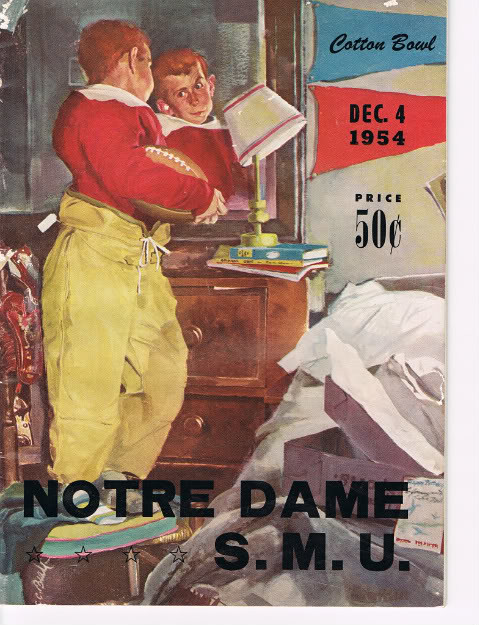This detailed depiction illustrates a vintage drawing resembling a Norman Rockwell painting, dated December 4, 1954. The scene centers on a young, red-haired boy with prominent ears, standing on a yellow and green step stool in his cluttered bedroom. Gazing intently at his reflection in a wall-mounted mirror, he holds a football in the crook of his right arm. Dressed in a vivid red jersey and yellow pants with a white drawstring, he appears absorbed in the moment.

Behind him, a wooden dresser cluttered with books and a night lamp adds to the room's disarray. On the wall to the right, two pennants are prominently displayed: a blue one reading "Cotton Bowl" and a red one noting the date "December 4th, 1954." Below these, the price "50 cents" is clearly marked. At the bottom of the image, in bold black capital letters, the names of the competing teams, "Notre Dame" and "S.M.U.," are inscribed. Additionally, four stars adorn the bottom left corner, providing further detail to this nostalgic and richly detailed composition.